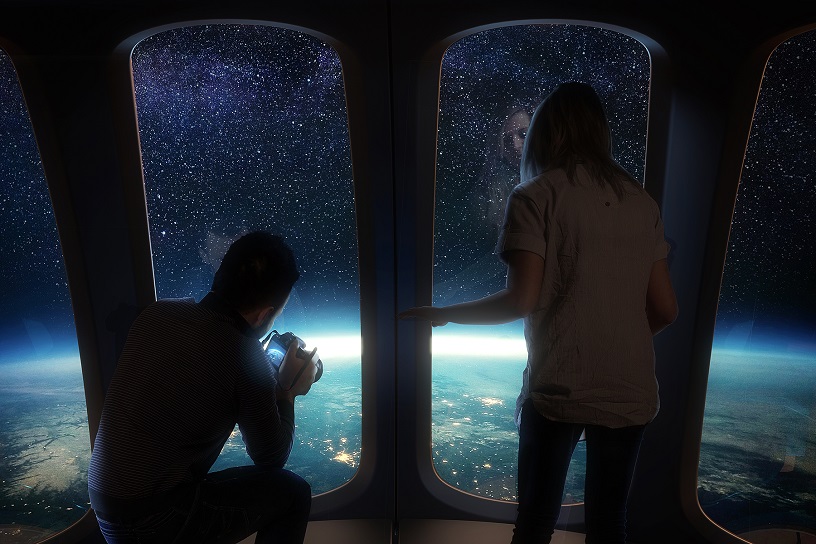In this striking image, we see two individuals within a futuristic or cinematic scene, likely from a movie or video game, emphasizing the unreal aspect of the depiction. They are situated in a dark, high-altitude or space environment, distinguished by a building or spacecraft with four tall oblong windows framed by narrow pillars. 

On the right stands a woman, her left arm extended as she gazes out the window at a distant planet. She is dressed in dark pants and a white or off-white t-shirt. To the left, a man is crouched on one knee, leaning to his right with a digital camera in his right hand, capturing the stunning view of Earth. Dressed in a blue sweater and jeans, he looks intently at the camera screen that displays the image of Earth.

The view outside the windows showcases the semi-circle of a planet in the bottom third of the image, illuminated by city lights that hint at life below. The top two-thirds of the scene is filled with the vastness of space, dotted with stars and hints of a purple galaxy, lending an ethereal quality to the dark surroundings.